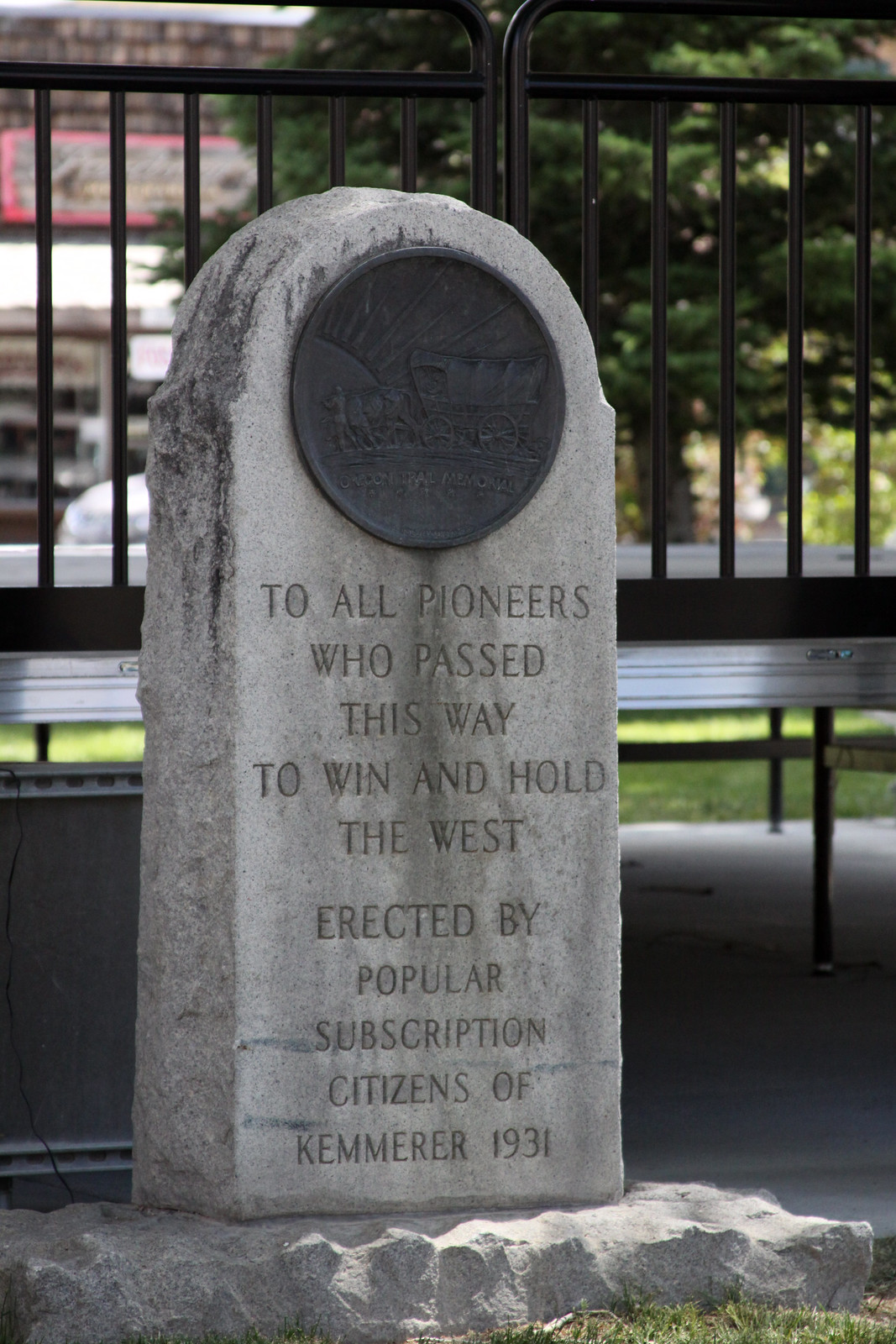The photograph captures a historic scene centered around a gray stone marker with an arched top, prominently situated in the middle of a grassy field. The gravestone features a large dark gray metal engraving at the top, depicting a stagecoach being pulled by horses. Below the engraving, the inscription reads, "To all pioneers who passed this way to win and hold the West, erected by popular subscription citizens of Kemmerer 1931". Surrounding the stone marker is a black metal rod fence, suggesting a defined historic or memorial site. The backdrop includes verdant green grass, a large tree, and distant buildings and a bridge, all under the clear midday sky, emphasizing this open-air park setting. The array of colors in the image spans green, gray, black, silver, pink, purple, and brown, reflecting the diverse elements of this evocative historic location.